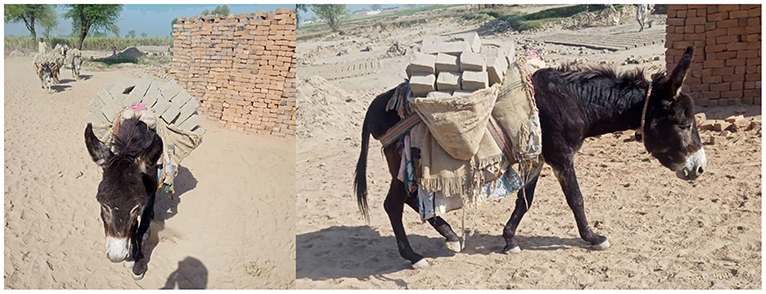This image features two side-by-side photographs of a working donkey, possibly the same animal, captured from different angles in a desert-like, hazy environment. The donkey is blackish-brown in color with prominent big ears and a white muzzle. In the left-hand picture, the donkey is seen from the front, showcasing its face and ears, while visibly carrying a load of beige or grayish-white bricks on its back. This donkey, along with two others in the background, is set against a backdrop of scattered bricks, hinting at a construction site, perhaps of a brick wall. The distant scenery includes palm trees and a patch of the blue sky, indicating a hot, arid climate. The right-hand picture provides a side view of the same donkey, emphasizing its burden and the simple cloth or saddle attached to its back for carrying the load. The donkey appears to be moving slowly and methodically, embodying the steady nature of a hardworking pack animal.